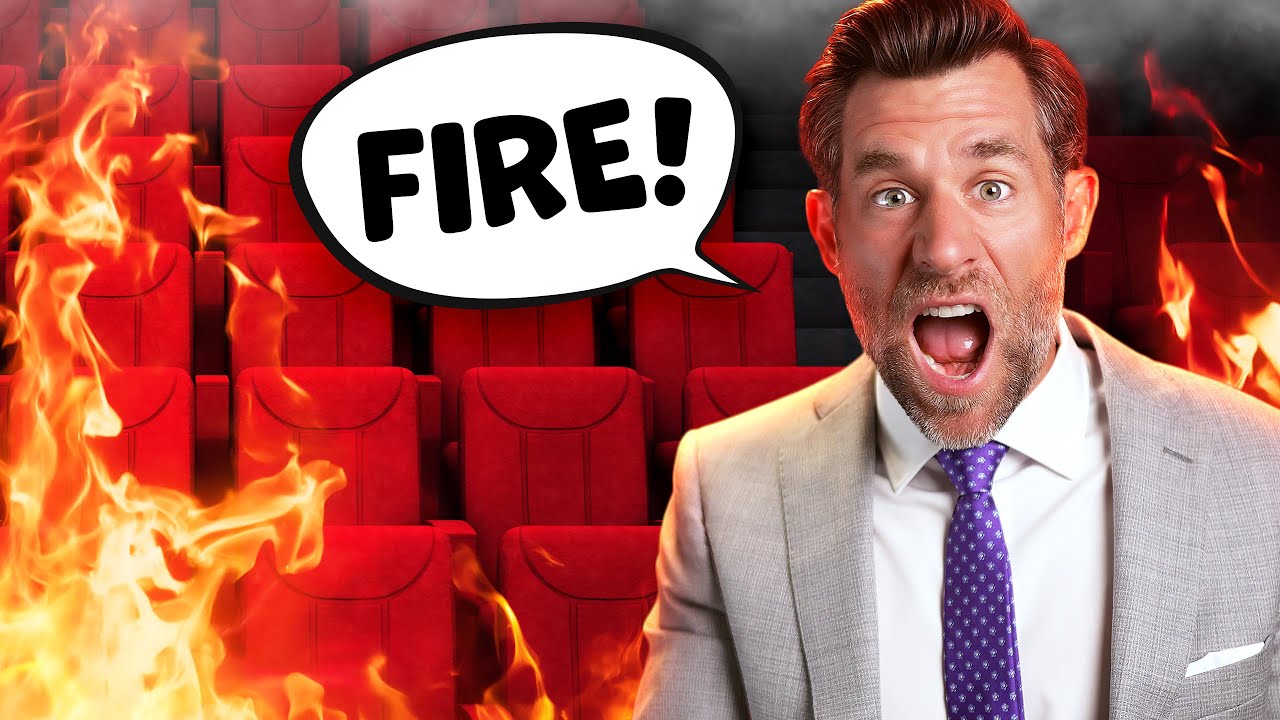The image depicts a theater room engulfed in flames, with fire visible on both the left and right sides. The theater features many red, cushioned seats arranged in ascending rows, each one higher than the previous. The seats have head cushions, armrests, and are divided into three sections on the back by two vertical stripes. On the right side of the image stands a man with a shocked expression, mouth open, and a speech bubble near him that says "Fire!" in black letters within a white circle. The man wears a light gray suit with a cream-colored shirt and a blue tie adorned with white star-like decorations. He has brown hair, slightly graying, and a beard that appears to be stubble or in the initial stages of growth. His hair is swept back from his forehead. The image looks digitally altered, giving it a cartoonish effect that includes the imposed fire and the speech bubble, suggesting the scene is designed to elicit amusement rather than depict realism.